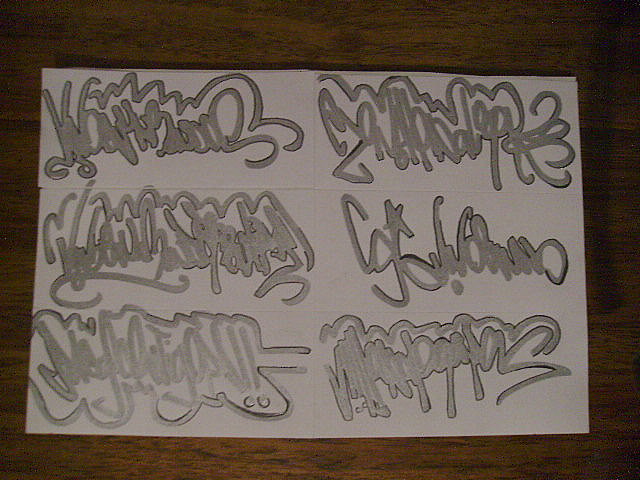This photograph captures a top-down view of six white rectangular pieces of paper arranged tightly together to form a larger square. These papers rest on a dark brown wooden table, with visible grain and centrally illuminated lighting that makes the surface appear lighter in the middle. Each piece of paper showcases intricate graffiti-like writing, rendered entirely in gray. The lettering, which bears a resemblance to cursive or an unknown script, features flourishes and bubble-like outlines around certain characters, enhancing its ornate appearance. The metallic and fine black marker strokes suggest different thicknesses, hinting that the same person created these elaborate, yet unreadable tags. Each piece of paper contains unique writings, ensuring no two are identical.